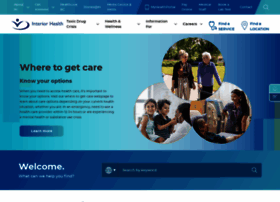Here is a detailed and cleaned-up caption for the image described:

---

This image depicts an extremely low-resolution screenshot of a health-related website. The webpage features a gradient background that transitions from teal blue to dark navy blue, with a lighter, white-tinged area slightly right of center. 

At the top left, a gradient-colored bar spans the width of the screen. Beneath this, a white navigation bar houses several options. Starting on the left, there is a blue logo depicting a stylized person with a swoosh below them, and to the right of the logo, the text "Interior Health" also in blue. The navigation bar includes four black-text options that are illegible due to the low resolution. 

To the right, there is text that possibly reads "Find a Physician" accompanied by a stethoscope icon, although it's not entirely clear. Further right, there appears to be a map pin icon with text beginning with "Find a," but again, the resolution makes it unreadable. In the top-right corner, there is a white magnifying glass icon, indicating a search bar nearby, though it lacks definition.

Below the navigation bar is a section that represents the lightest part of the screen, continuing with the teal-to-navy gradient. Central text reads "Where to get care," followed by "Know your options." Underneath this headline is a paragraph of dark gray text that is too blurry to decipher. 

Beneath the paragraph is a button with reversed gradient coloring, navy to teal blue from left to right. The white text on the button is mostly unreadable, possibly saying “Launch” something.

On the right side of the screen, three overlapping circles are arranged in a triangular formation, reminiscent of Olympic rings. Each circle contains a photo: the top circle shows two older individuals walking outdoors, possibly with a walker, amidst greenery and trees; the bottom left circle depicts a young girl and boy, likely interacting with a doctor in a lab coat; and the bottom right circle features what appears to be a medical professional in scrubs talking to a patient in a hospital bed. Both individuals in this last image seem to have darker skin and dark hair.

Further along the right edge, there is a vertical set of arrows; the upward arrow is on a teal background while the downward arrow is on a navy background. Just below this, there is a darker bar with white text starting with “Welcome," though the subsequent words are unclear. Adjacent to this section, a rectangular area hints at another search bar, but its low resolution leaves it indistinct.

---

This detailed caption aims to convey a thorough description of the webpage elements despite the low resolution of the original image.